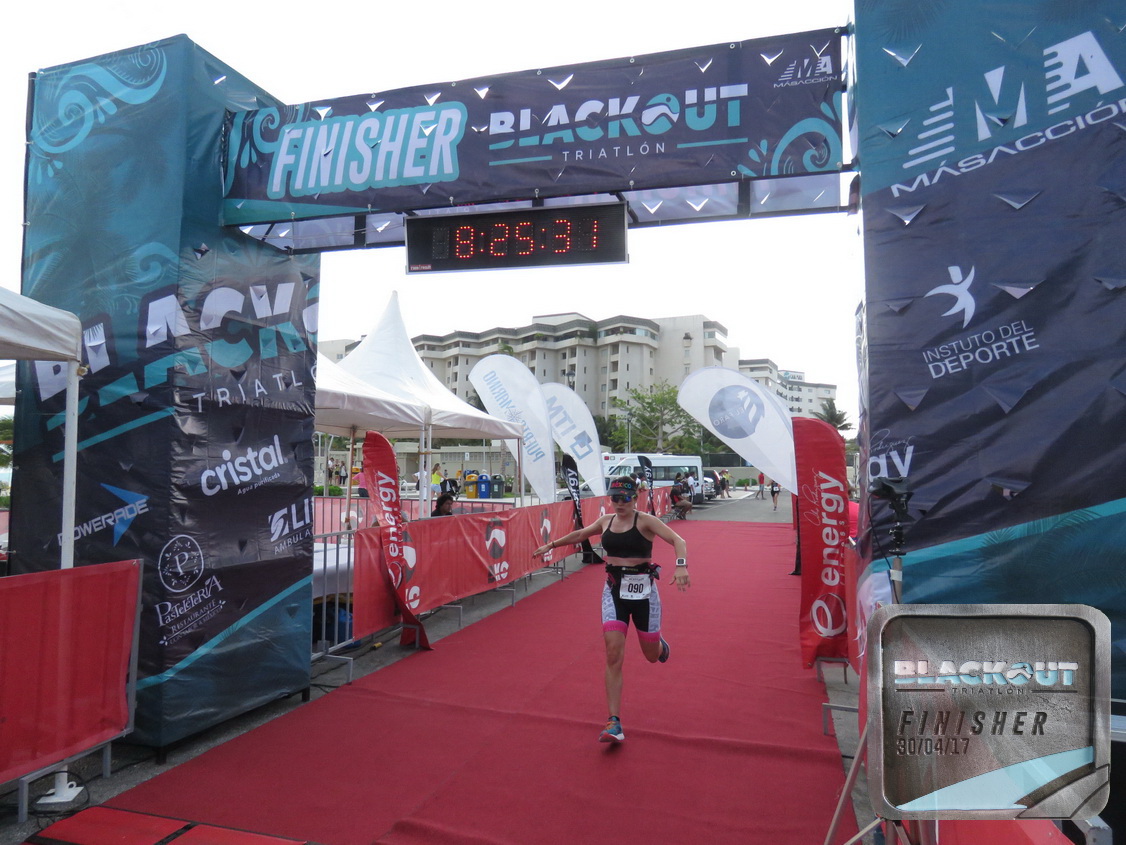This photograph captures the exhilarating moment of an athlete crossing the finish line at the end of a triathlon race. The scene is dominated by a prominent blue archway structure emblazoned with the text "Finisher Blackout Triathlon." Suspended from this structure, a display screen prominently shows the completion time of "8:25:31." The athlete, likely a woman clad in a short black top and black and gray shorts, sprints forward with her hands raised victoriously, showcasing the action of the moment. Beneath her feet is a vibrant red carpet marking the final stretch of the race. Flanking the running area are tents and boards featuring various advertisements, including a sign that reads "Black Beauty Finisher" and another with Spanish text "M.A. Masacuchillan Deporte." In the background, an apartment building looms, along with visible emergency equipment such as parked vans, highlighting the race's outdoor setting. The overcast sky adds a white hue to the atmosphere, completing this vivid depiction of the race's concluding segment.